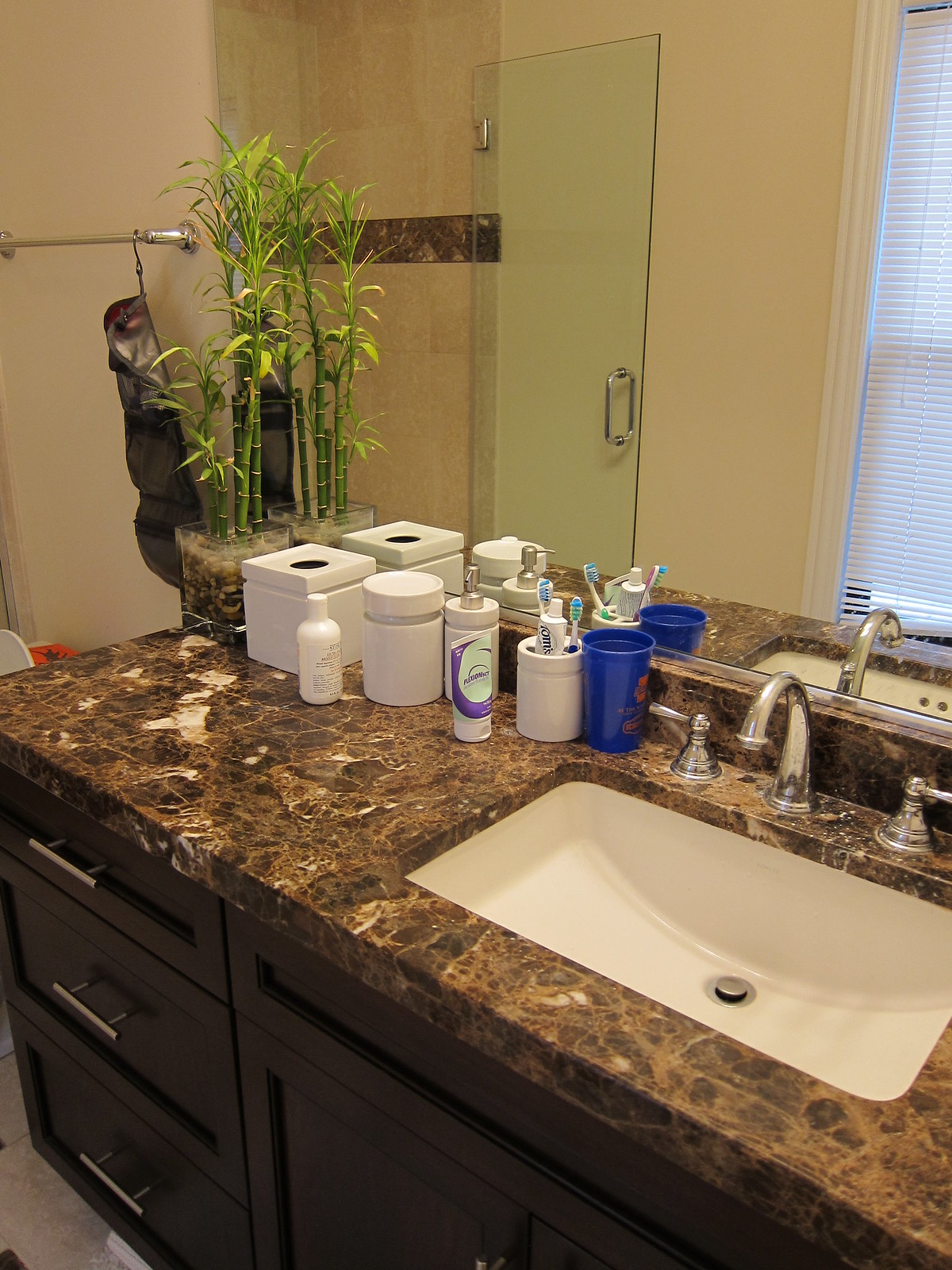In this detailed photograph, which is presented in portrait mode, we observe a close-up view of a bathroom sink and vanity area. The vanity unit features a rich, dark brown wooden front adorned with modern brushed nickel handles. On the left side of the vanity, three drawers are arranged in descending sizes: a small drawer at the top, a medium one in the middle, and a larger one at the bottom. Underneath the sink area, there are two partially visible cabinet doors – the top half of the left door and the corner of the right door.

The countertop is a striking dark chocolate marble with a busy white marbled pattern reminiscent of swirled s'mores, adding a complex visual texture. The sink itself is a modern, rectangular white basin, mounted beneath the countertop to ensure easy cleaning. Complementing the sleek sink design are shiny silver nickel-plated faucets with separate handles for hot and cold water, and a stylish gooseneck spout.

Atop the countertop, on the far left side, sits a clear glass square pot containing small bamboo plants anchored in decorative rocks. To its immediate right is an empty white plastic tissue box. Continuing from left to right, there is a small bottle potentially containing lotion or shampoo, though the label is indistinguishable. Beside it stands a white round canister, also without identifiable markings.

Next in line is a cylindrical silver soap dispenser that matches the faucet’s finish. Adjacent to that is a squat tube resembling a toothpaste tube, with a mint green background and a bright, deep purple swirl pattern. A white toothbrush holder filled with grooming items – including a tube of toothpaste and two toothbrushes with blue and green bristles – is placed next. Completing the lineup is a blue plastic cup, emblazoned with an unreadable orange logo, which appears to be empty.

A large mirror is mounted behind the sink, reflecting parts of the bathroom. In the background, a towel holder, the lid of a toilet with the seat up, and an orange item resting on the toilet tank can be seen.